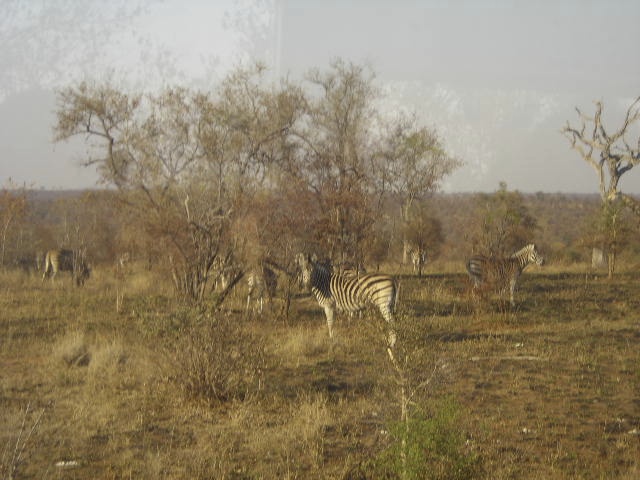This faded, grainy photograph captures a scene on a parched African plain, likely taken with an old-style camera on a sunny, hazy day. The ground is predominantly covered with brown, dead grass with sparse patches of greenery, indicating a very hot climate. Numerous zebras are scattered across the landscape, their tan and black striped bodies creating a striking contrast against the dry, barren terrain. One prominent zebra in the center faces the camera directly, while others are seen grazing or milling about, some partially obscured by scrubby, leafless trees. In addition to the zebras, there are vague, large brown animals, possibly giraffes, wandering off into the distance. The background features low hills or mountains under a blue, slightly cloudy sky. The trees are noticeably sickly, with most either bare or sporting dying leaves, contributing to the overall sense of a harsh, sun-beaten environment.